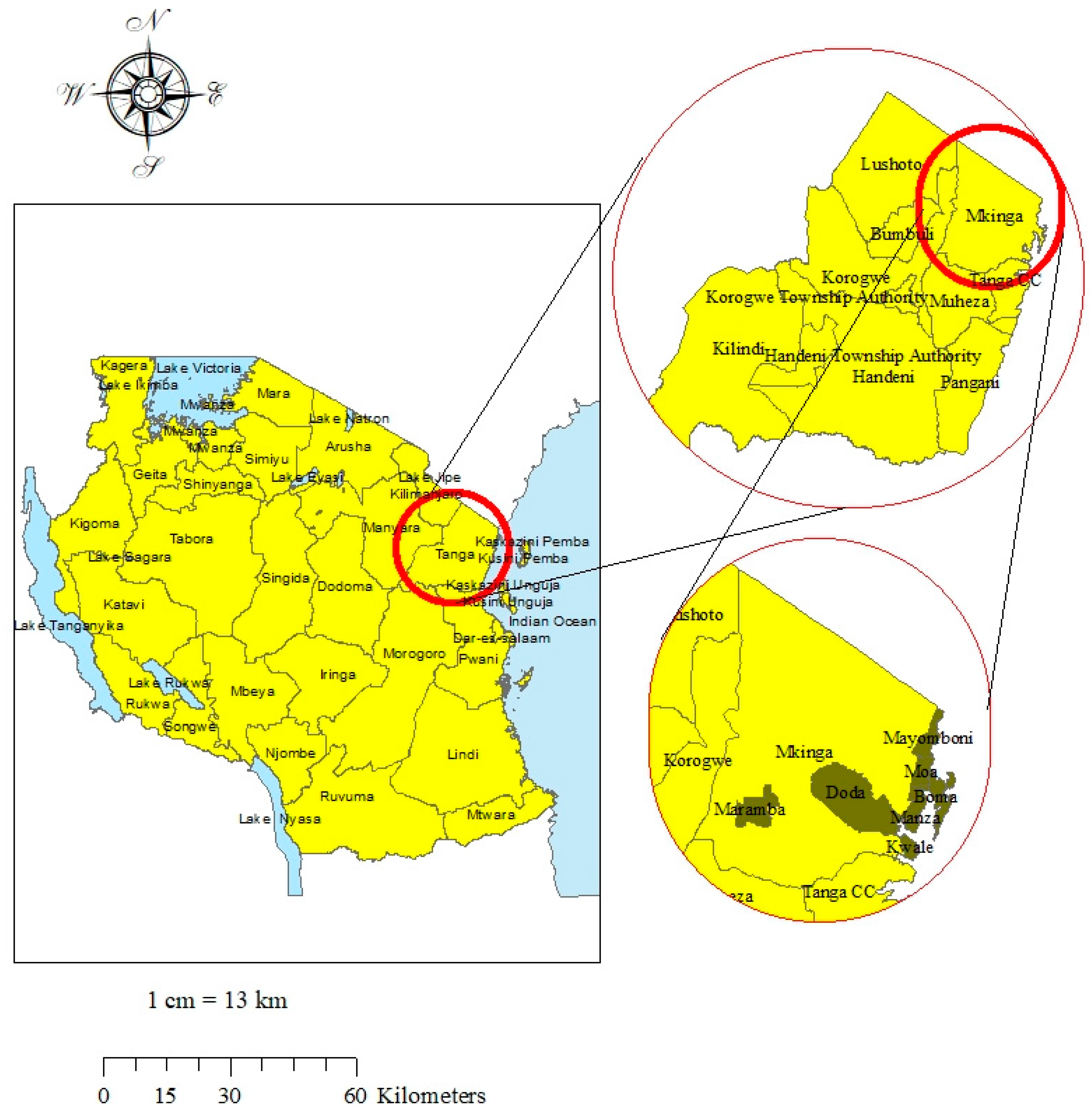This image is a detailed map of a region in Africa, prominently featuring Lakes Tanganyika and Victoria, with the Indian Ocean also indicated. The map shows various cities including Goma, Tabora, Katabi, Mbeya, Dodoma, Iringa, Morogoro, Tanga, and Makinga. It is color-coded with yellow indicating land and blue denoting water bodies. The map is outlined in black with a compass rose displaying north, south, east, and west directions. 

There are two red-circled areas on the map. The first red circle encompasses the easternmost part of the map, which is then enlarged to reveal smaller towns and villages, providing greater detail of this segment. In this area, Tanga is a notable mention. The second red circle highlights Makinga, and this area is further zoomed in under the initial enlargement to show close-up details, potentially indicating areas of interest or concern though the specific reasons for highlighting are unclear.

The map includes a scale that states one centimeter equals 13 kilometers, with a graphical representation ranging from 0 to 60 kilometers. Overall, the map is very detailed, providing a structured illustration of the region with notable emphasis on specific areas through magnified insets.